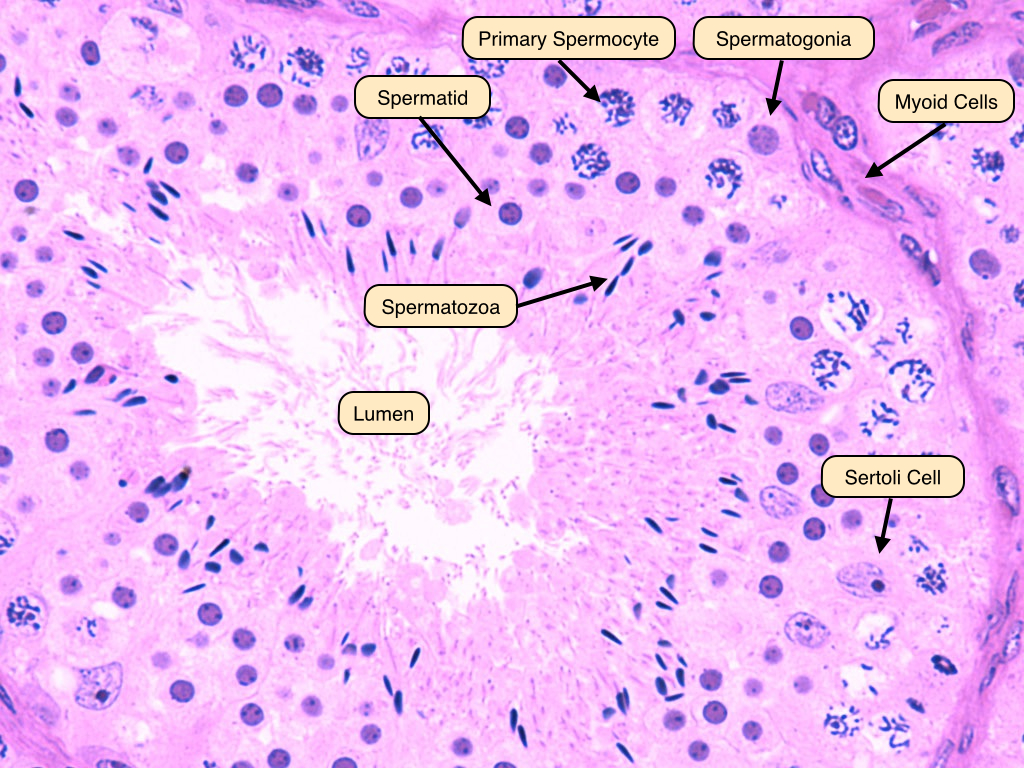The image is a detailed rendering of various cell types, predominantly in shades of pink and purple, with intricate markings and labels. This artistic, yet scientific illustration features a central white area labeled "lumen." Surrounding this are numerous cell structures denoted with tan, rounded labels and black arrows pointing directly to the respective cells. Key identified cells include:

- "Spermatid": positioned towards the top of the illustration, depicted with discernible cell walls.
- "Primary Spermatocyte": adjacent to the spermatid, illustrated as a dark blue sunburst shape.
- "Spermatogonia": near the primary spermatocyte, lighter in color.
- "Myoid Cells": located further right, depicted as oblong structures.
- "Spermatozoa": described as dark blue streaks, situated to the right of the lumen.
- "Sertoli Cell": a light-colored cell with a darker center, found below the spermatozoa.

Overall, the image combines a mix of cell shapes, including dots, oblong pieces, and lines, over a base of pink and purple hues, providing a comprehensive view of the intricate relationships between different cell types.